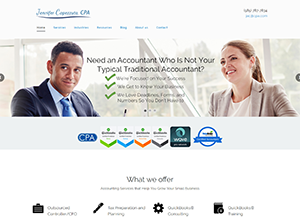Screenshot of a Blurry Website with Overlay Content:

In this screenshot of a website, captured from a computer monitor or laptop, the image is noticeably reduced in size and slightly blurry. In the top left corner, there is the website’s name in blue text underlined by a darker blue line, although the text is indiscernible. Below the website name are six or seven clickable options, with one in black and the others in light blue, though these too are unreadable. The top right corner also contains some illegible text.

The main focus of the image is a central headline: "Need an accountant who is not your typical traditional accountant," followed by three lines of content with green check marks, which are similarly blurry and unreadable. Below that, there is a section titled "What We Offer," featuring several black text options that are also out of focus.

The image prominently features a man and a woman. The man, with short black hair, is dressed in a blue suit jacket, a light blue collared shirt, and a bright blue tie. He is smiling and looking to his left. The woman, with brown hair pulled back, is also smiling. She is wearing a light brown suit jacket over a white shirt. The overall image conveys a professional and friendly atmosphere, despite the blurriness.